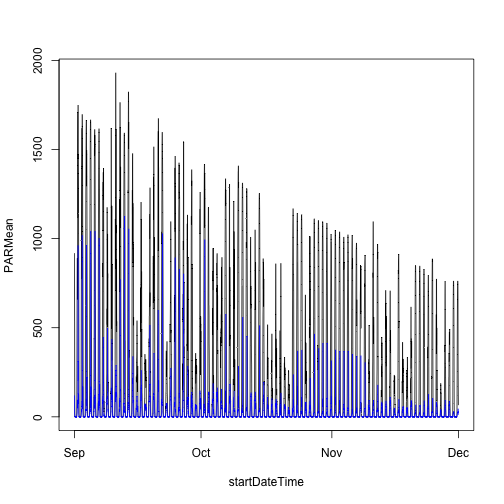This image displays a highly detailed bar chart characterized by thin blue, black, and gray bars across a square graph. The bars begin tall on the left side and trend downward towards the right, presenting a fluctuating pattern of highs and lows. The vertical axis on the left, labeled "PARMEAN," scales from 0 at the bottom up to 2000 in increments of 500. Along the bottom horizontal axis, months are abbreviated as SEP, OCT, NOV, and DEC, corresponding to the "Start Date Time." The chart reveals detailed, compressed data for each day within these months, where the values rise and fall in a recurring pattern, indicating high peaks and low troughs in activity or measurements consistently across the timeline.